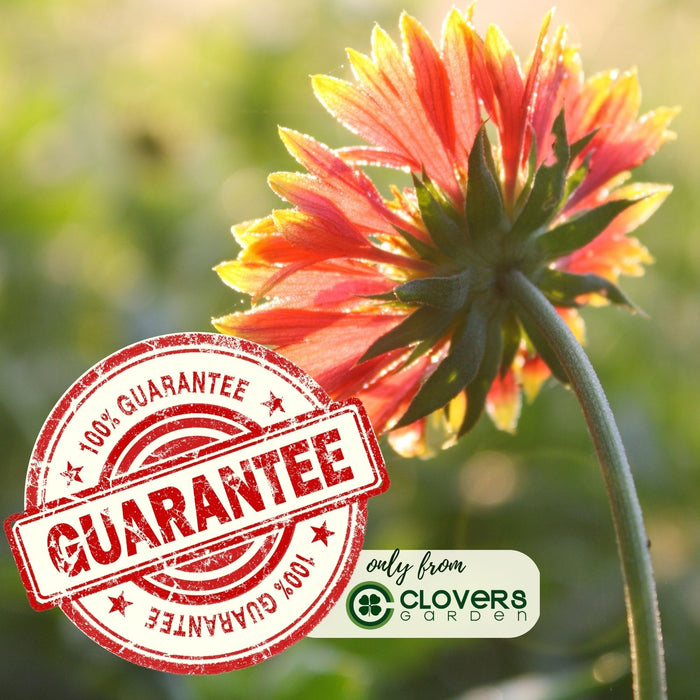This close-up photo captures a spectacular flower from an uncommon perspective—the back side. Dominating the right side of the image, the flower features a vibrant blend of colors. The green stem supports the bloom adorned with small green leaves at its base. The petals are densely packed, slender, and exhibit an array of hues: red, pink, orange, with yellow tips. Although the bloom is fully open, the photo angle doesn’t reveal its interior.

On the left side of the picture, a notable red and white stamp reads "100% Guarantee," prominently displayed at the top and in the middle with the word "guarantee" in large letters. Additionally, there is an upside-down and repeated mention of "100% guarantee." Another sign, which features the text "only from Clover's Garden," is also visible. This leafy product label is set against a milk-colored background with green text, completing the scene.